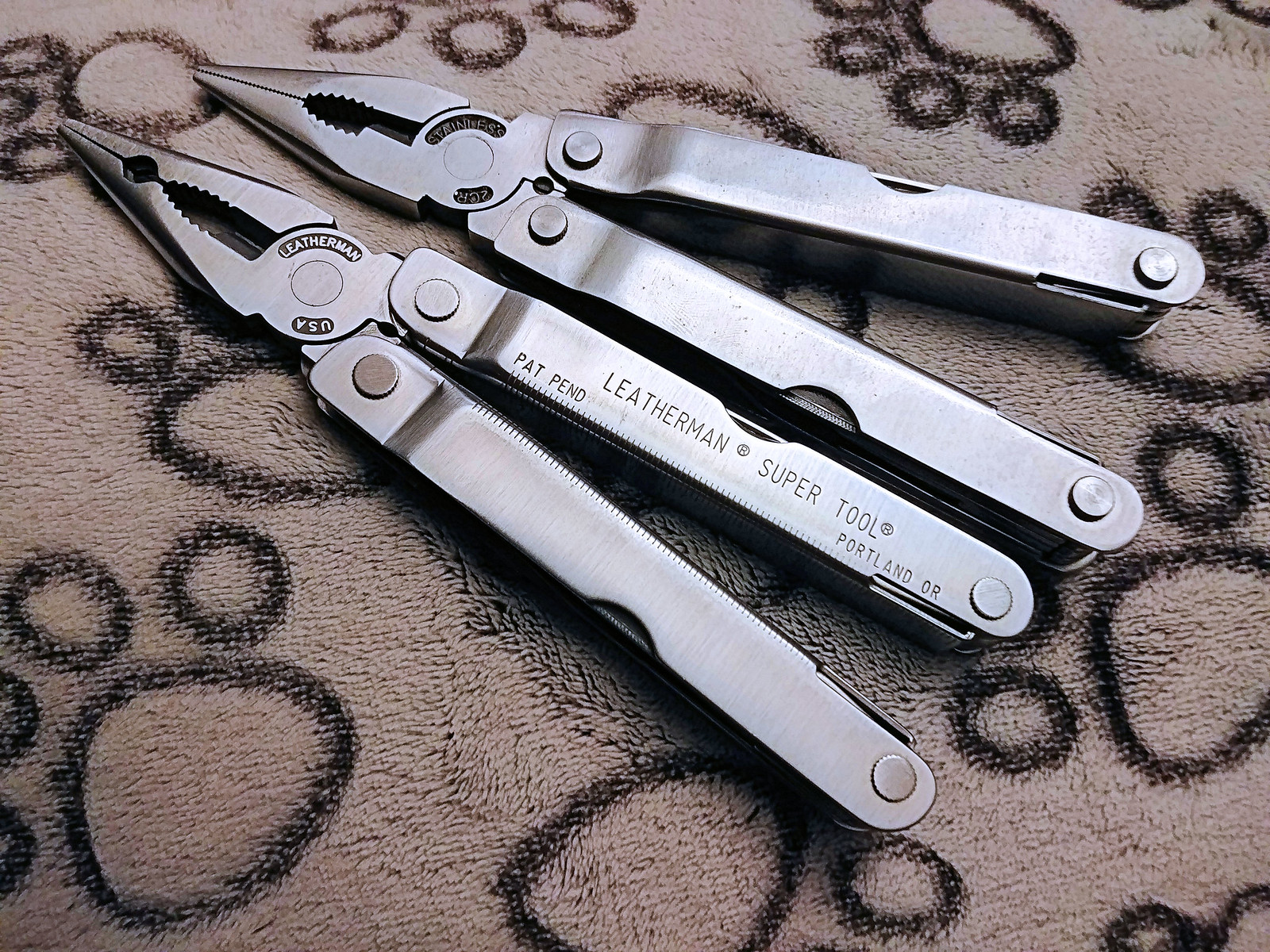In this detailed photograph, two almost pristine tools are laid out on a brown, decorative surface adorned with what appear to be black bear or dog paw prints. The tools are identified as needle-nose pliers with metallic handles. The pliers rest with their handles in the lower right corner of the image, while their heads point towards the upper left.

The tool in the lower part of the frame is distinctly etched with several details: "Leatherman Super Tool," "Pat. Pend.," and "Portland, OR" with "USA" displayed near the pivot. The upper tool, although similar in design and functionality, lacks any inscriptions.

Both tools gleam with a silver finish and feature handles that suggest additional functionalities similar to a multi-tool or pocketknife. The meticulous arrangement and clarity of the features indicate that these are high-quality, durable tools intended for versatile use.